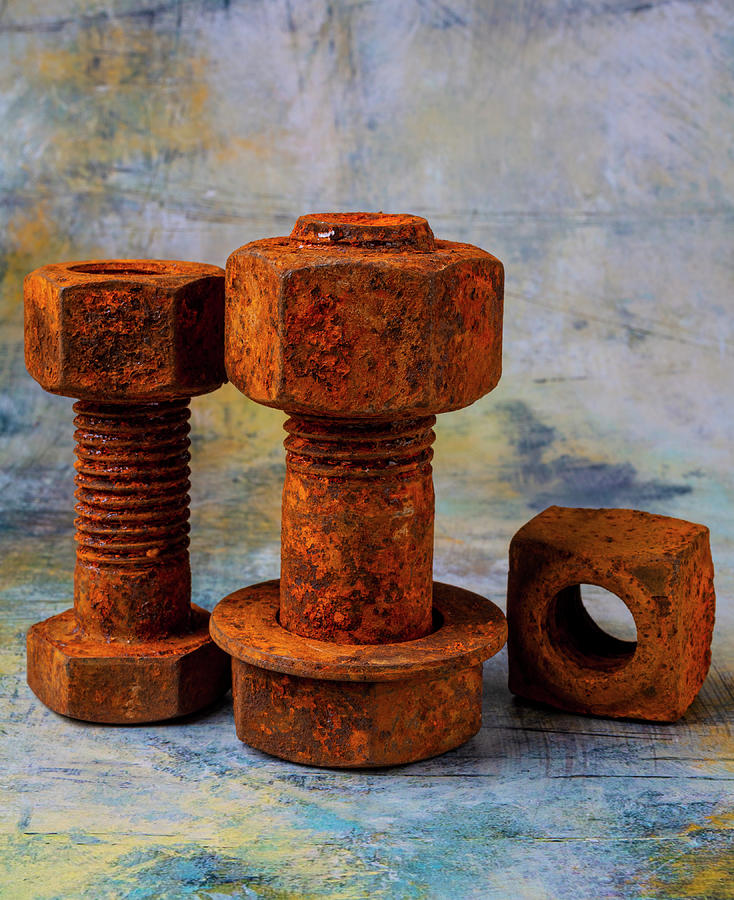The photograph depicts a meticulously composed art piece featuring two prominently rusted bolts, each with a hexagonal nut threaded onto them, and one of the bolts, thicker than the other, also adorned with a washer. The rusty elements are arranged on an artistically scratched and paint-splattered wooden surface, suggesting an artist's studio backdrop. Both bolts are positioned standing on their heads, with their threaded ends pointing upwards. To the right, complementing the composition, sits a distinctive square nut, adding to the diverse geometric interplay of shapes. The background features an abstract convergence of blue and yellow hues with earthy brown tones peeking through, enhancing the artful and industrial aesthetic of the entire setting.